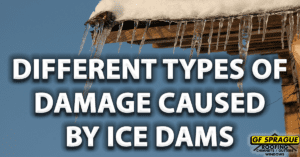The image features an advertisement for GF Sprague roofing, showcasing the effects of ice dams on roofs. It has a blue sky background and prominently displays white block text in three lines: "different types of damage caused by ice dams." The photograph captures a close-up section of a roof, partially covered with a white sheet of snow, and several large, clear icicles hanging from the edges. In the bottom right corner, a yellow rectangle contains the black text "GF Sprague" with the word "roofing" below it, along with a black outlined triangle representing a roof. The colors in the image include shades of blue, white, yellow, black, and various browns from the roof structure. This professional image likely originates from a roofing website and serves to illustrate the potential roof damage that can occur due to ice dams, emphasizing the need for professional roofing services.